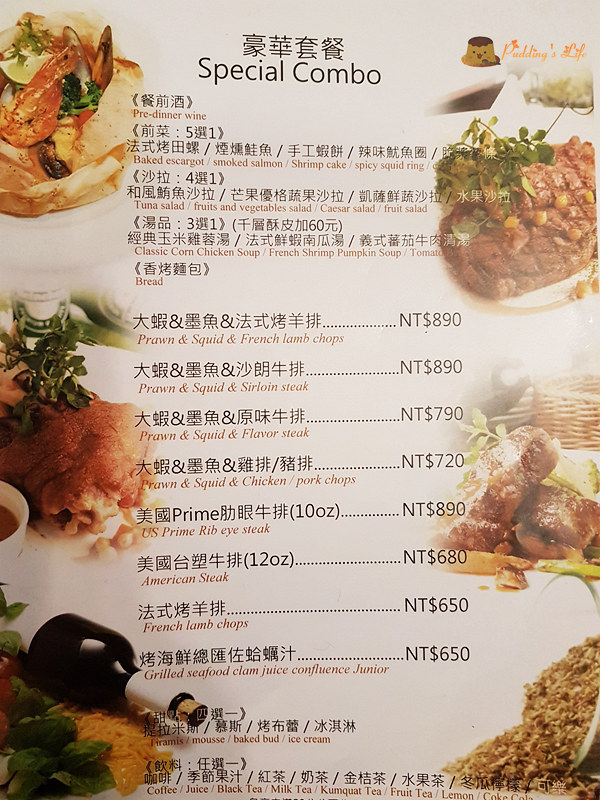The image showcases a detailed menu from an Asian restaurant, prominently featuring both Asian characters and their English translations. At the top, there's a section labeled "Special Combo," with Asian lettering above it. Each menu item is displayed with a corresponding Asian script above their English names. Among the listed dishes are pre-dinner wine, baked escargot, smoked salmon, shrimp cake, spicy squid rings, tuna salad, classic cornbread chicken soup, bread, prawns, and squid French lamb chops. Each item is neatly organized into its own section with prices ranging from NT$6.50 to NT$8.90.

The background of the menu is primarily white, adorned with various pictures of the food items on the page. Visible images include a shrimp dish, bread, a steak dish, and a bottle of wine beside what might be pasta or shredded cheese. In the top right corner, the phrase "Puddings Life" is written in orange, accompanied by a cute image of a smiling pudding dessert. The bottom right corner features another image that appears to depict grains.